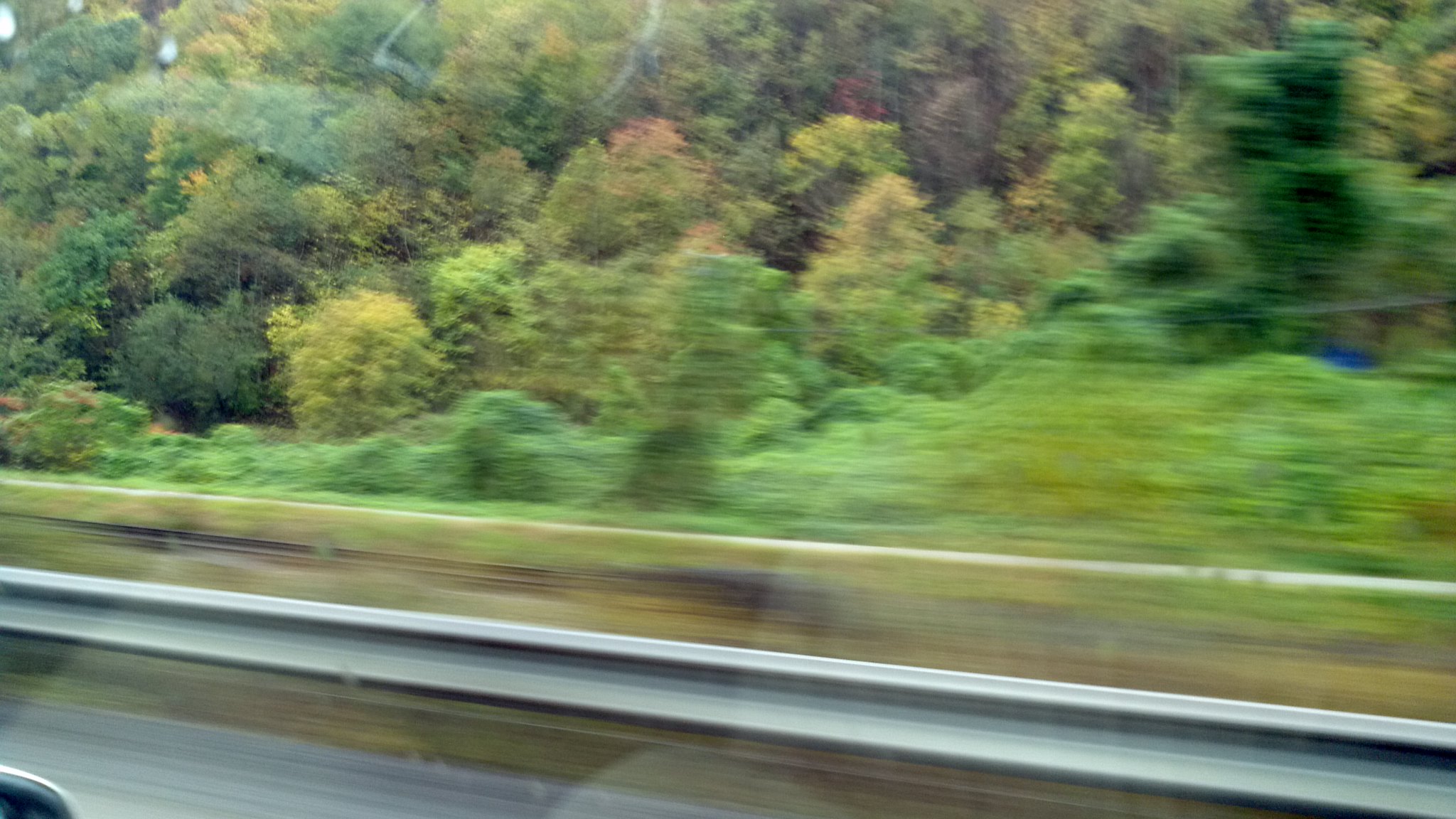The photograph captures a blurry scene, taken from a large moving vehicle, likely a bus or train, evidenced by the wide, undivided window frame. The motion blur distorts the image, smearing details into indistinct lines. In the reflection on the window, dim outlines suggest the presence of vehicle seats or a center console, and the vague shape of a person wearing a light-colored top. The landscape outside features an array of lush greenery, including tall trees, short bushes, and varied foliage, with hints of red leaves suggesting an autumn setting. You can see the road's metallic crash barrier and a median, indicating the vehicle is traveling along a highway. Among the greenery, a blue object—possibly a tarp or bucket—is faintly visible but unidentifiable due to the blur. The sky appears overcast, adding to the image’s indistinct and somewhat gloomy ambiance.